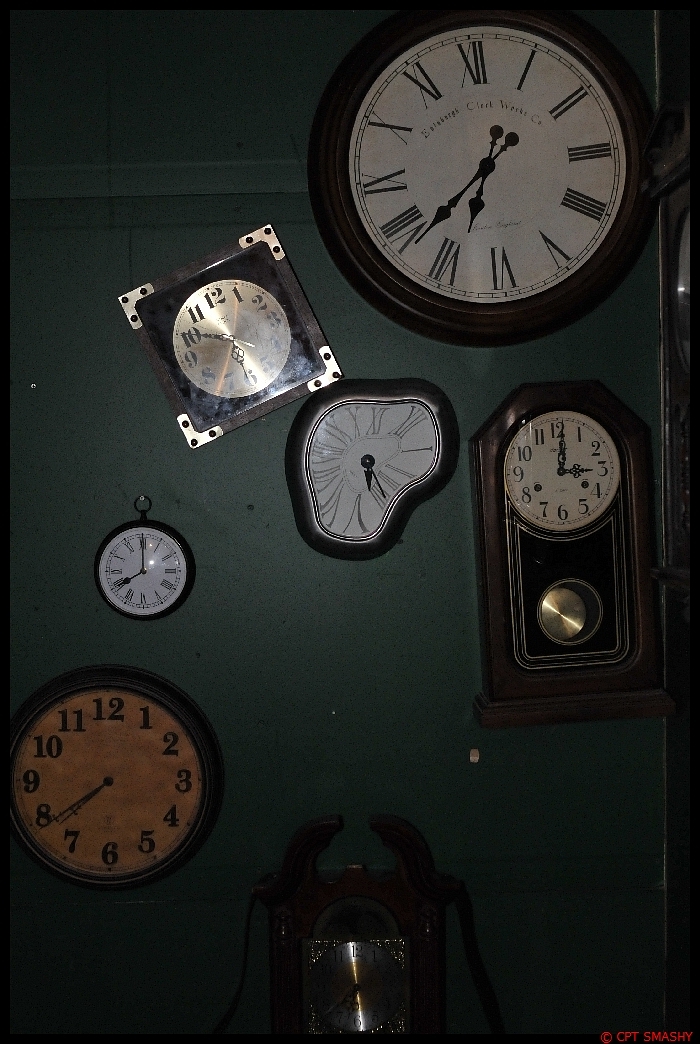In this image, six (and possibly seven) clocks are displayed against a green wall in a vertical arrangement. At the bottom center of the image, partially shrouded in darkness, sits a clock with a discernible metallic base. On the lower left side is a clock resembling those found in schools, with a small wall clock positioned just above it. At the right center, a formal wooden wall clock with a pendulum adds an element of sophistication. To the left of this clock is an almost triangular-shaped clock, angled towards the upper left. Above this, slightly angled, is a metal clock featuring a brass face set within a square mount. Completing the collection, at the upper right, is a traditional wall clock with a wooden frame, a white face, black hands, and Roman numerals, enhancing the eclectic mix of timepieces on display.